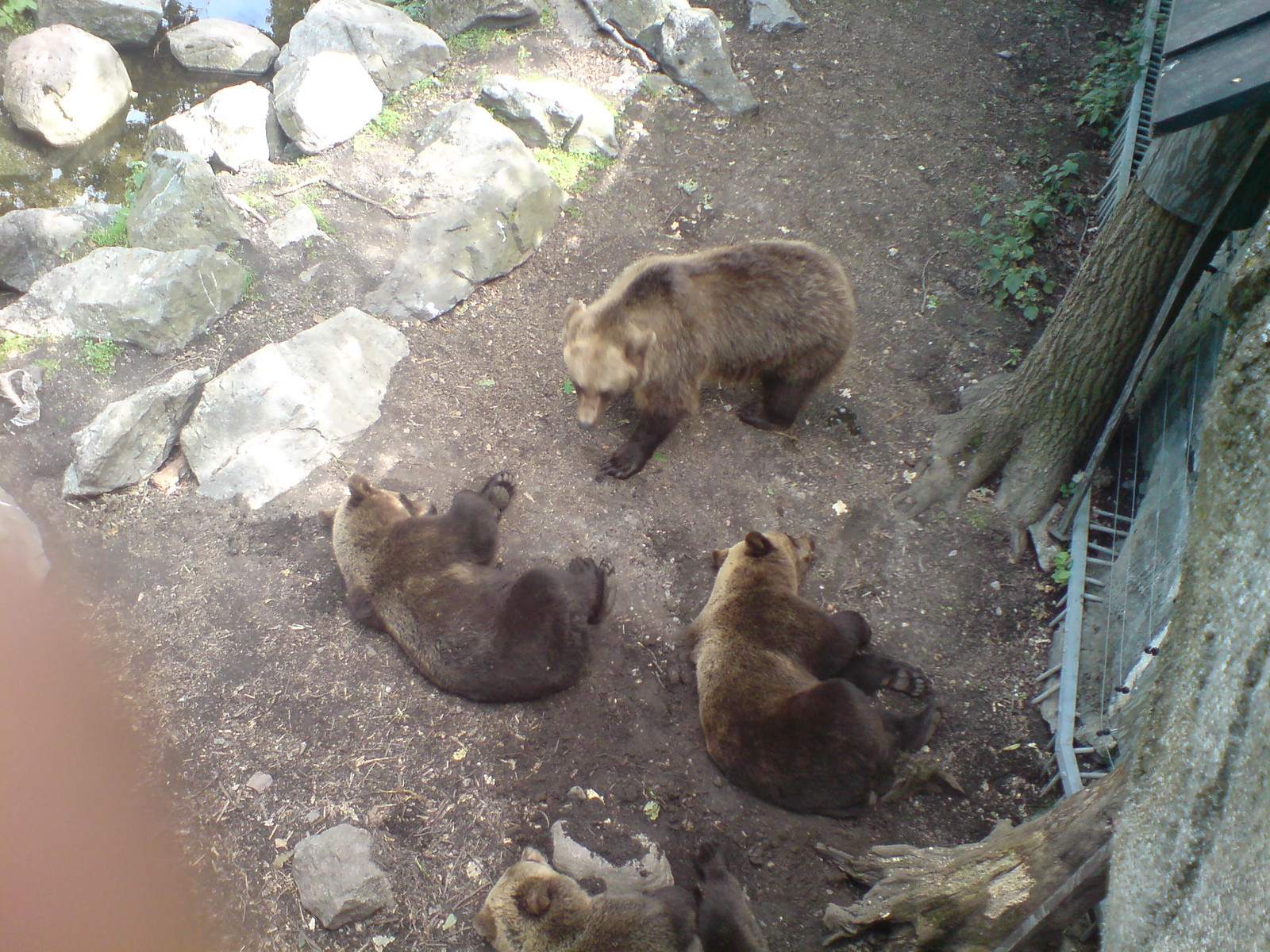The image is an aerial bird's-eye view of a zoo enclosure housing four brown bears. The terrain consists of a mix of brown and gray dirt with patches of green vegetation, particularly towards the right side. The upper left corner showcases large rocks interspersed with smaller pebbles and bits of greenery. Two trees, rooted firmly in the ground, create a naturalistic setting, and a metal fence runs between and past them, hinting at human-made structures within the enclosure. 

Three bears are lying down, seemingly asleep. One of these bears rests on its side, with darker haunches and a lighter head. Another, positioned slightly to the left, also lies on its side, displaying a grayish-brown coloration with a similarly shaded head. A third bear is distinguished by its dark shoulder and arm and is positioned on its side too, with lighter hues on its head and back.

The fourth bear is walking towards the others, showcasing a contrast between its light brown body and almost white head, possibly preparing to lie down. The bottom right corner of the image reveals brownish water flowing onto the ground, accompanied by a lone rock. A slight blur affects the bottom left corner, likely from a finger obstructing the camera lens.